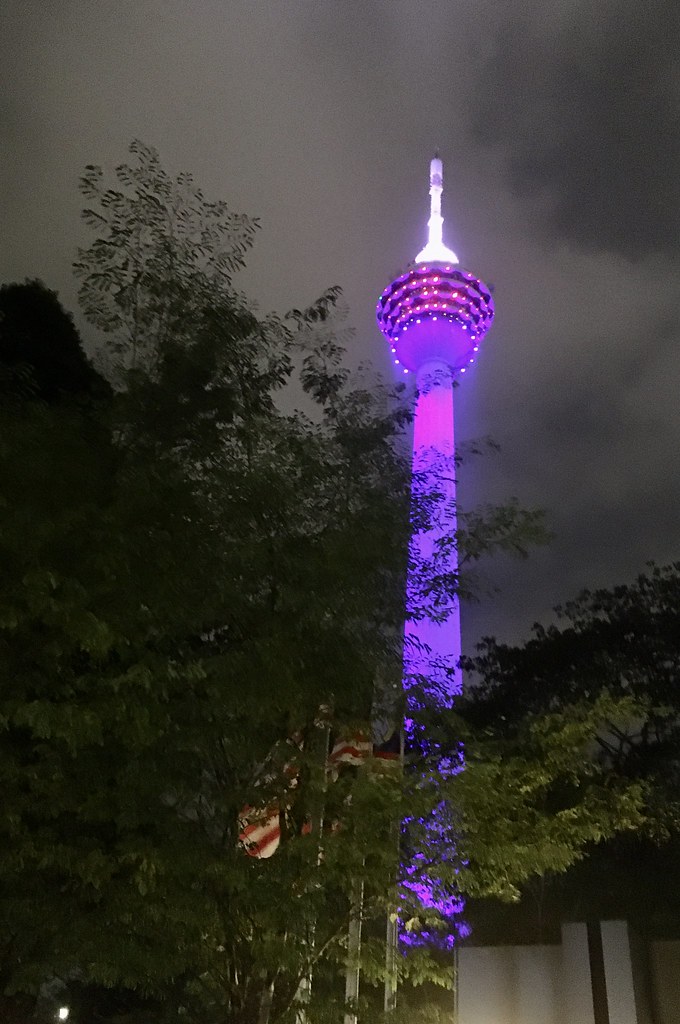In this nighttime image, the central focus is a tall tower resembling Seattle's Space Needle, prominently illuminated in vibrant purple and pink hues. The tower has a distinct rounded section near the top that glows with these colors, while the apex features a white pole. Tiny yellow lights can be seen at its peak. The sky is dark and cloudy, adding a dramatic backdrop. Surrounding the base of the tower, there are green-leaved trees, partially obscuring the view. To the left of the tower, multiple flagpoles with American flags are visible, showcasing the red, white, and blue colors alongside the star pattern. Additionally, a white wall is discernible at the bottom center of the image, contributing to the detailed night scene.